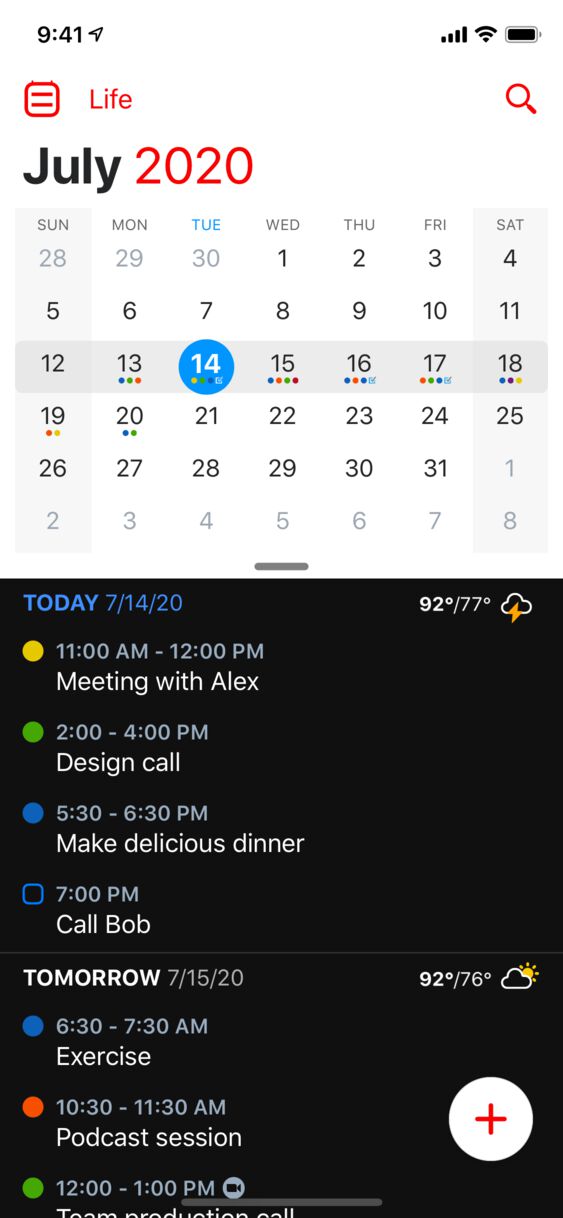In the upper right corner of the image is an icon depicting a full battery and a cell phone, both filled with a black color. To the left of this icon is the time displayed as "9:41." Below the time is a square symbol enclosing two horizontal red lines representing the signal strength, and next to this is the word "life" in red text, accompanied by a magnifying glass icon to its right. The month "July" is written in black text, with "2020" in red text beside it.

Beneath this section is a calendar grid displaying the week from Sunday to Saturday. The month begins on a Wednesday (the 1st) and ends on a Friday (the 31st). The only date circled is Tuesday the 14th, distinguished by a blue circle.

Further down, there is a section labeled "Today" with the date "7/14/2020" and the temperature forecast of "92 degrees." Below that, an agenda lists:
- "11 to 12," a meeting with Alex,
- "2 to 4," a design call,
- "5:30 to 6:30," a reminder to make a delicious dinner,
- "7 p.m," a call with Bob.

The following section, labeled "Tomorrow," includes the date "7/15/2020" with scheduled activities:
- "6:30 a.m. to 7:30 a.m.," exercise,
- "10:30 to 11:30 a.m.," a podcast session.

Beside the "Tomorrow" section is a red circle.